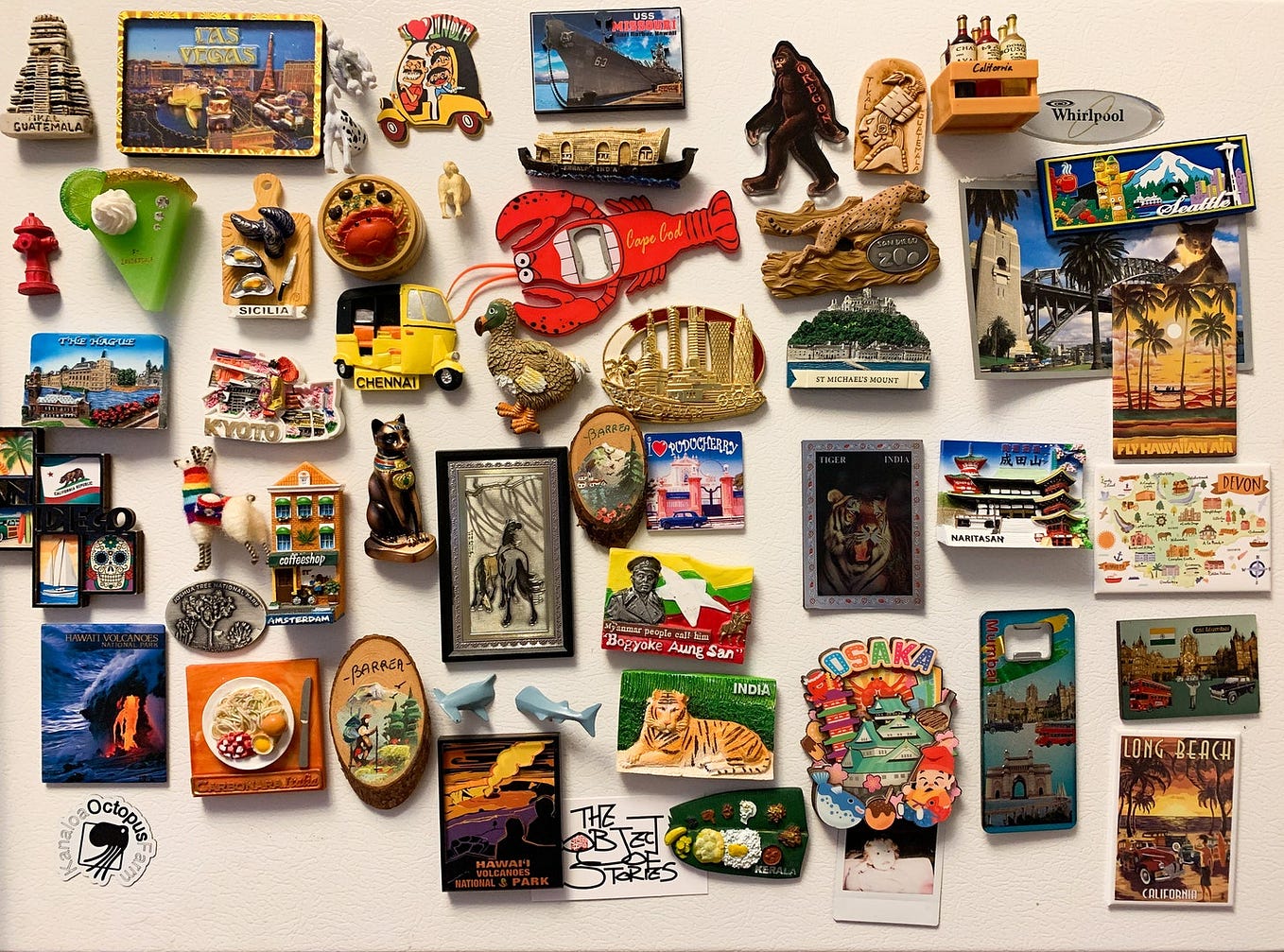This photograph captures a vibrant and eclectic collection of refrigerator magnets from various countries, artfully arranged on a Whirlpool fridge. The display features a myriad of magnet types, including animals, food items, iconic landmarks, and cultural symbols. Among the highlights are a two-piece hammerhead shark magnet that appears to be diving into the fridge, a whimsical lobster bottle opener from Cape Cod, and a Bigfoot magnet representing Oregon. 

Notable international magnets include:
- A tiger from India.
- A pyramid from Guatemala.
- Clams on a chopping board from Sicilia.
- Old cars on the beach from Long Beach.
- Various food items like a key lime pie and a fried egg.
- A depiction of the USS Missouri battleship.
- A koala bear and a "Fly Hawaiian Air" magnet featuring palm trees and the ocean.

Additional colorful magnets showcase scenes from cities such as Kyoto, Chennai, and Mumbai, alongside a fire hydrant, flags, and landmarks from Las Vegas, California, Seattle, and Osaka. Some magnets bear humorous or culturally significant images, though a few depict outdated and racially insensitive caricatures, such as a Japanese baby in Osaka and a crowded car labeled "I love India."

The collage also includes non-magnet elements such as a small sign stating "Best of Stories" and a "canola octopus farm" advertisement, adding to the diverse visual tapestry of this magnet collection.